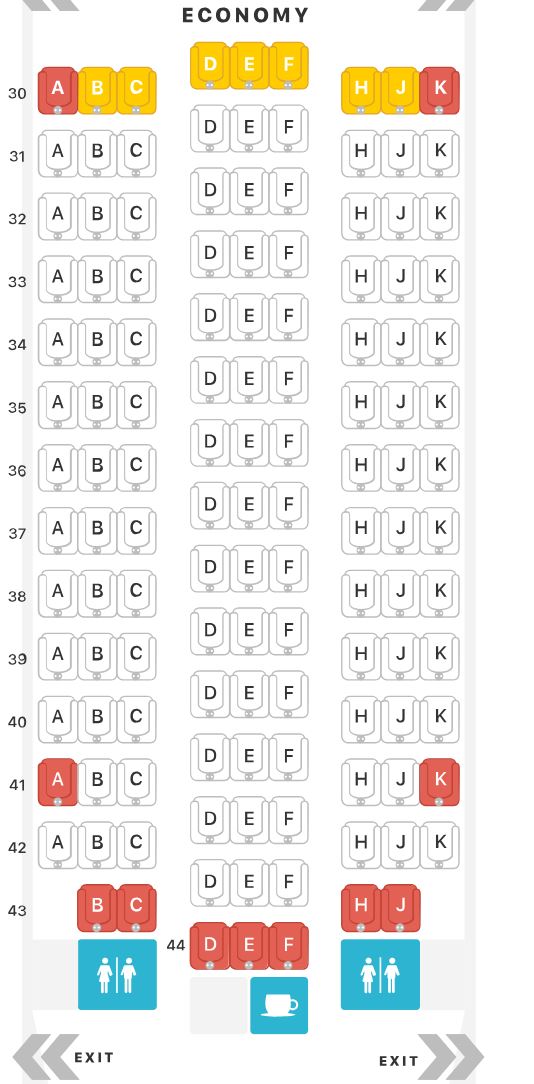The image is a screenshot of an airplane seating assignment webpage or application, predominantly featuring white, black, orange, red, blue, and gray colors. At the top of the page, the word "ECONOMY" is prominently displayed in bold, black, uppercase letters. The seating chart begins at row 30 and extends through row 43, arranged in a 3-3-3 configuration separated by two aisles. 

In row 30, seats labeled A and K are marked in red, indicating they are likely occupied or unavailable. Seats labeled B, C, D, E, F, H, and J are marked in yellow, suggesting they are available for selection. This pattern of labeling continues throughout the chart, with most seats already assigned. Only a few seats remain unassigned.

Key facilities are also indicated on the seating chart: lavatories are marked in blue at the bottom of the image, and a compartment labeled "COFFEE" is situated at the back of the plane, also in blue. This detailed layout helps passengers easily identify available seats and onboard amenities.